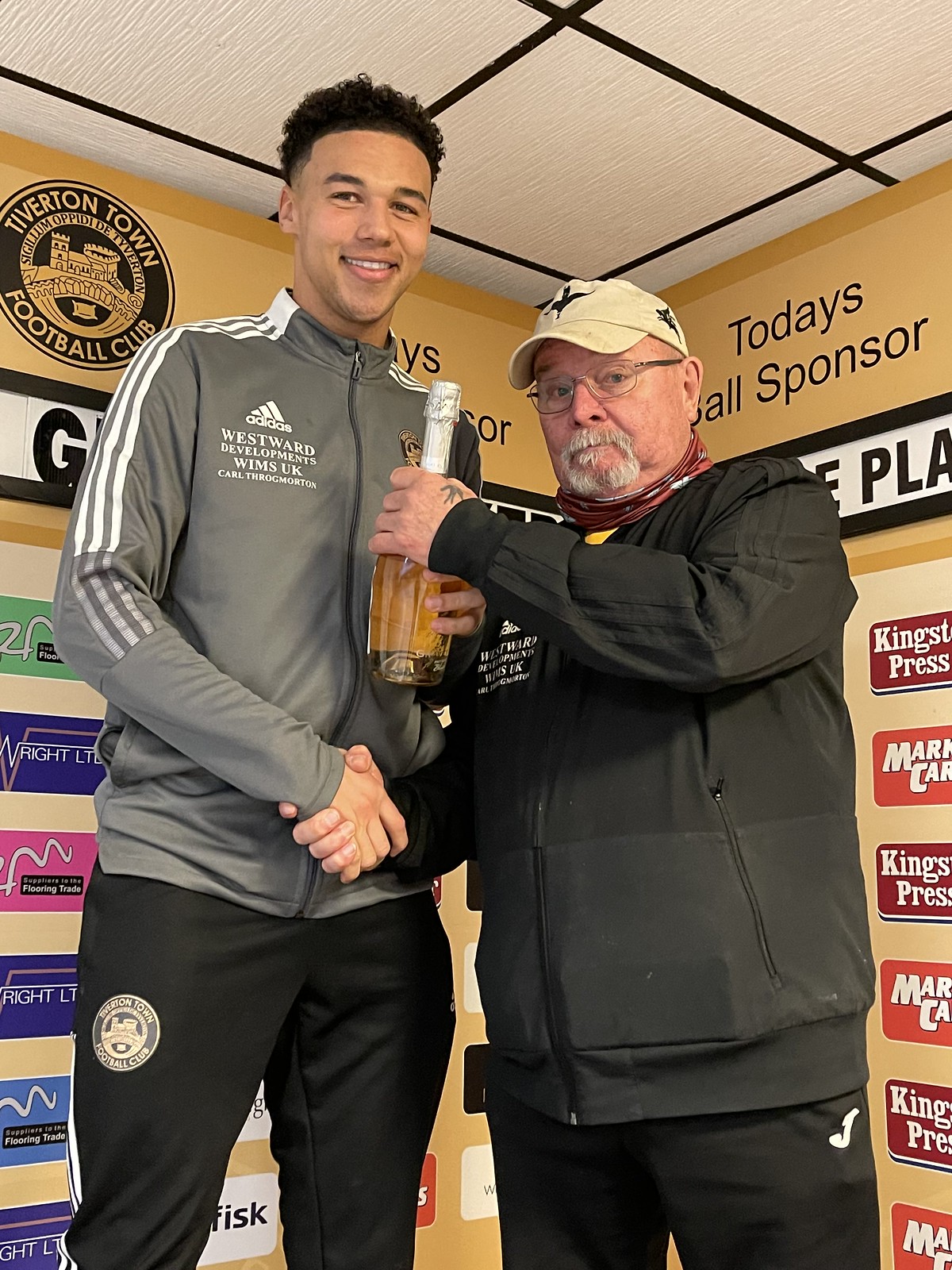In this image, two individuals are posing side by side, engaged in a handshake, while simultaneously holding a wine bottle together. The person on the left is a tall, younger man with dark hair and eyes, attired in a gray Adidas tracksuit jacket adorned with white stripes running down its sides. The left front of his jacket features the text: "Adidas, Westward Developments, WIMS, UK, Carl Thrugmorton." He pairs this with black tracksuit pants that also have white stripes on the sides. Standing to his right is a significantly shorter, older gentleman with gray hair, a beard, and a mustache, wearing glasses and an ivory-colored baseball hat with a kangaroo emblem. He is dressed in a black windbreaker, zipped up, along with black pants. The backdrop reveals a yellow-beige wall displaying signage for Tiverton Town Football Club and a section dedicated to 'today’s sponsor,' surrounded by various other sponsor logos.